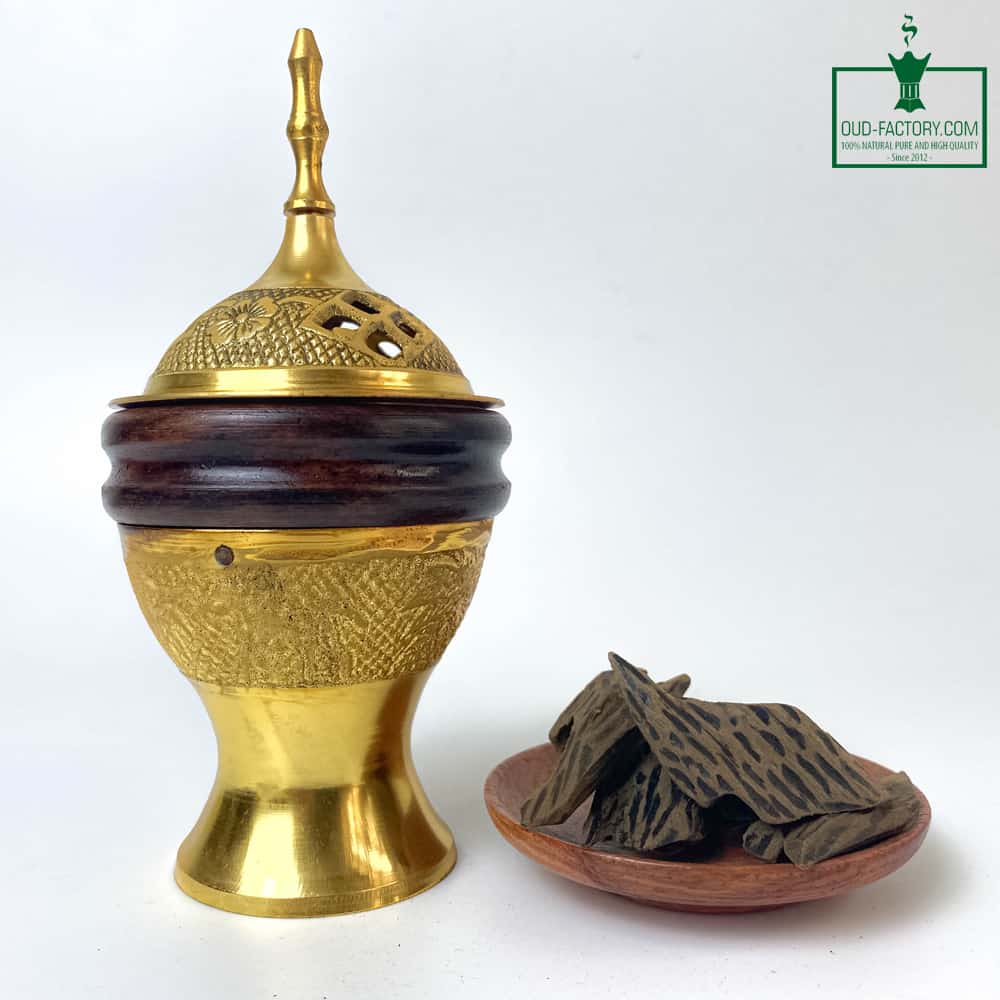The image showcases a golden, ornate incense holder or urn with an egg-like shape and a built-in stand, featuring a brown wooden middle section. It has a detachable, indented lid atop its golden structure, which gives it a distinctive, orthodox appearance. To the lower right of this incense holder, there is a small, shallow wooden bowl containing chunks of medium-toned brown incense that resemble tree bark, interspersed with black indentations. The background of the image is gray, and in the upper right corner, a green rectangle logo reads "OUD-FACTORY.COM, 100% natural, pure, and high quality since 2012," with an illustration of an urn or incense burner emitting smoke.